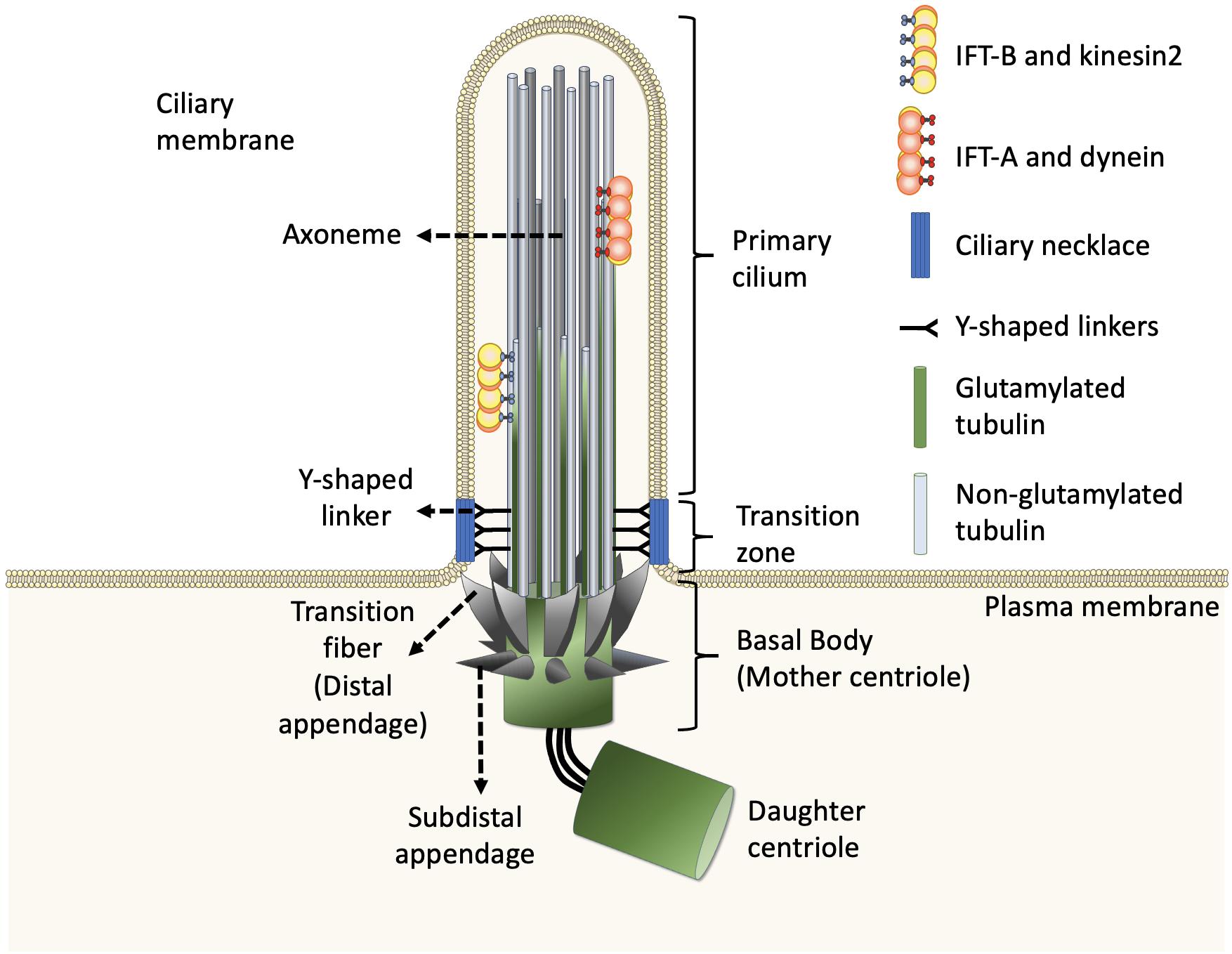This detailed diagram illustrates the structure of the ciliary membrane. At the bottom, there is a green cylinder referred to as the "daughter centriole," connected by various transition fibers and appendages to another green cylindrical base termed the "mother centriole" or "basal body." This base is characterized by spikes known as transition fibers, distal appendages, and subdistal appendages. Rising from the basal body is an array of metal rods labeled as the "axoneme," with Y-shaped linkers at their base connected to the plasma membrane. The rods are adorned with both red circles labeled IFT-A and dynein, and yellow circles labeled IFT-B and kinesin-2. A circular array of rods is encircled by a string of lights forming an arch. A beige band, identified as the ciliary membrane, traces the outer structure and is marked at the top of the tube as the "primary cilium." Notably, two blue rods within this structure are identified as ciliary necklace pieces. The legend on the top right helps identify these components, while the upper left corner labels the complete structure as the "ciliary membrane." The diagram's various annotations and color-coded parts provide a complex but thorough visualization of this intricate cellular structure.